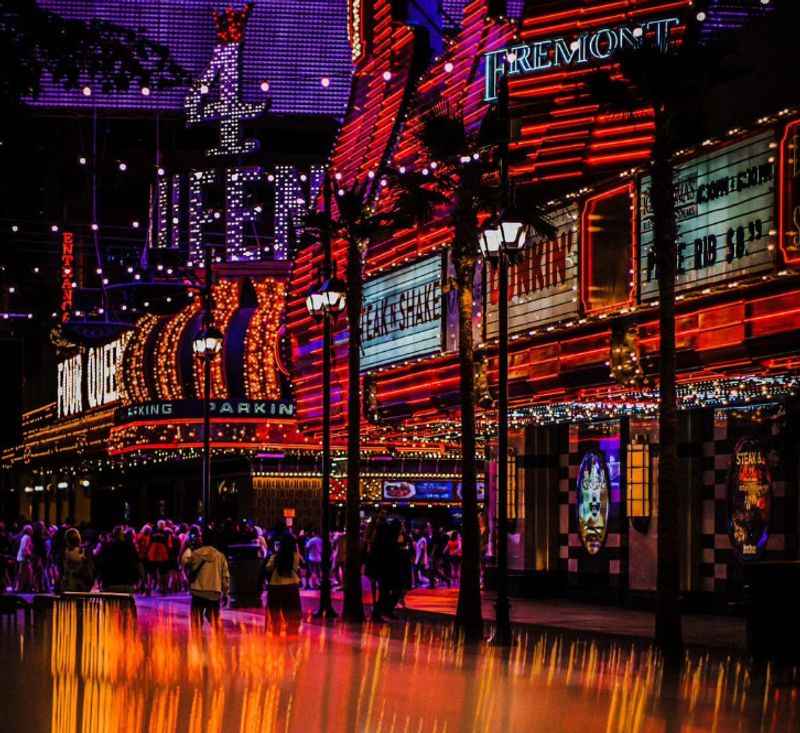This image captures a vibrant nighttime scene in what appears to be downtown Las Vegas, specifically on Fremont Street. The focal point is the prominently lit Four Queens hotel and casino, whose neon signage appears in multiple locations: horizontally and vertically in dazzling purple and yellow lights. The area is bustling with pedestrians walking along a concrete sidewalk in front of various establishments. Signs for well-known eateries like Dunkin' and Steak 'n Shake add to the festive, touristy atmosphere. Notably, a sign advertising prime rib for $58.99 suggests prime dining options available in the vicinity. The image is dominated by an abundance of neon lights, including a large, bright sign for "Fremont" and another for "Parking," casting a colorful glow over the scene and enhancing the distinctive Las Vegas feel. The bottom of the picture features a blur of orange lights, likely from streetlights or signage, contributing to the scene's dynamic, lively ambiance.